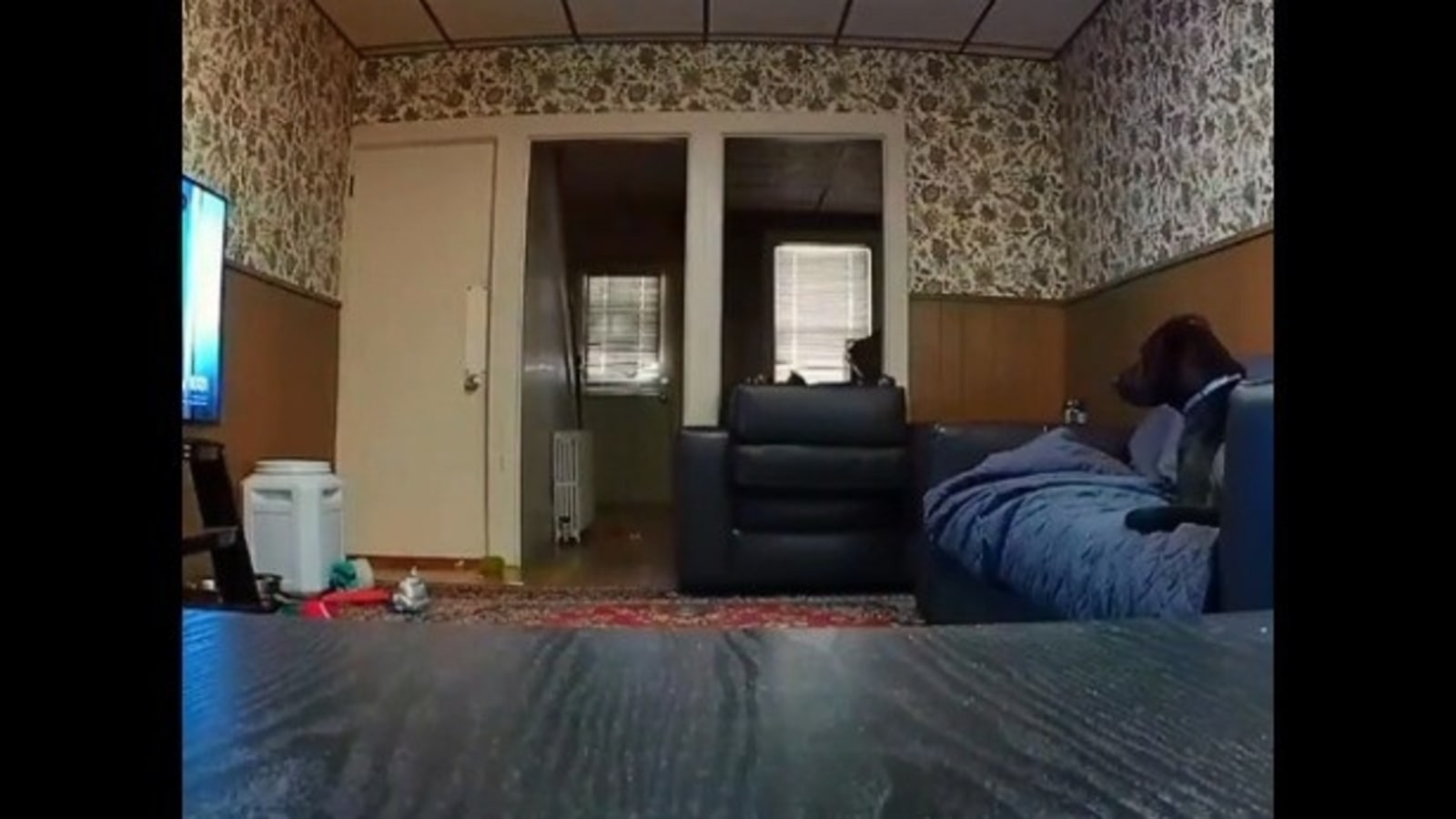In this image, a black dog wearing a grey collar is seated to the right on a blue leather couch, which is covered with a dark blue fabric. To the left of the dog is a black leather chair, partially obstructing a white-framed doorway that leads to another room. Another doorway, possibly leading to a stairwell, is also visible. The scene includes a window next to a white radiator on a brown wooden floor. A third door, closed and cream-colored, is also present. High on the left wall, there's a white, rounded canister. The upper portion of the walls features brown and whitish-patterned wallpaper, while the lower portion displays brown wood paneling. The ceiling is adorned with white and black checkered markings. Additionally, a black metal stand supports a black-framed television, which shows hints of white and blue on its left side. In the foreground, the shot appears to be taken from a black wooden table with distinctive wood grains. A red patterned carpet with a brown outline partially covers the floor.